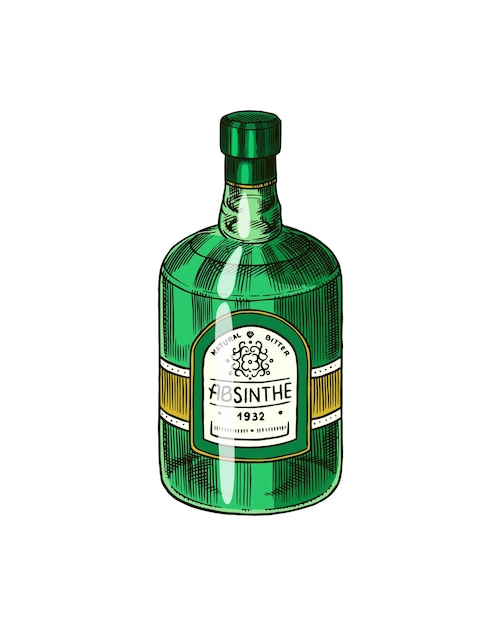This detailed illustration depicts a vintage-style bottle prominently labeled "Natural Bitter Absinthe 1932." The glass bottle has a light green, translucent hue and features a distinct green cap with two points. A decorative logo, featuring a floral design, is centered on the bottle's green label. Adding to its charm, a light brown band with vertical black lines and a white border encircles the center of the bottle. The overall design, including the gold ring around the bottle, is evocative of early 20th-century artistry and emphasizes the timeless allure of absinthe.